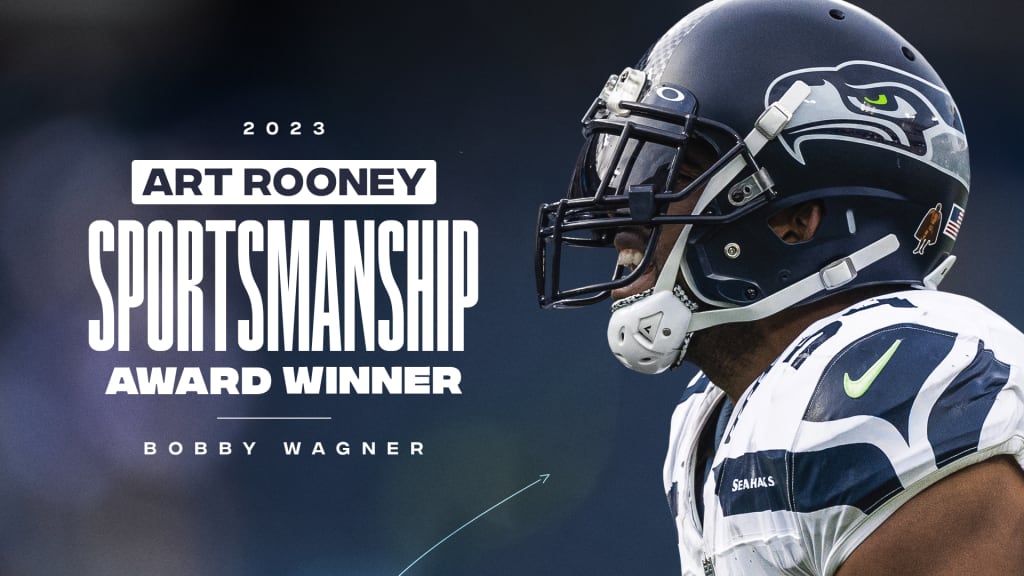This image is a promotional graphic designed for social media or sports websites, highlighting the 2023 Art Rooney Sportsmanship Award winner, Bobby Wagner. The focal point of the image is a dynamic photograph of Bobby Wagner, a Seattle Seahawks player, located on the right side of the composition. Wagner is depicted in an expressive pose, his mouth slightly open as if he is roaring or celebrating. He wears a Nike-sponsored white jersey with blue and green accents, and a blue helmet bearing the fierce-looking Seahawk logo. His helmet includes a visor, giving the appearance of sunglasses over his eyes. The background is a dark blue, completely blurred out to emphasize the subject and the text. 

On the left side of the image, there is bold, white text announcing the award. The words "2023 Art Rooney Sportsmanship Award Winner Bobby Wagner" are displayed with "Sportsmanship" being the most prominent and largest text, followed by "Art Rooney" in blue text. The design features a varied font size to draw attention to key elements, ensuring that "Bobby Wagner" and "2023" are also highlighted, albeit in smaller text. The overall layout and color scheme focus on creating a celebratory and attention-grabbing visual that clearly conveys Wagner's achievement.